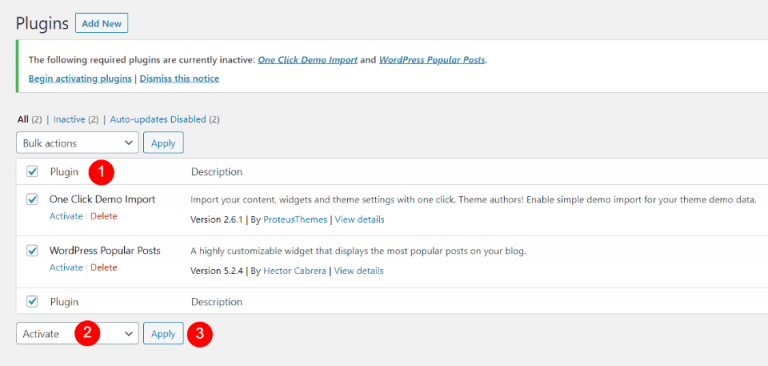At the top left corner of the screen, the title "Plugins" is prominently displayed, with a blue "Add New" button situated next to it. Just below this section, a warning message alerts the user: "The following required plugins are currently inactive: One Click Demo Import and WordPress Popular Posts." The message is accompanied by links to either activate the plugins or dismiss the notice. 

The current view displays a list of all installed plugins, with a red number "1" circled, seemingly drawn on the screen to indicate the initial step. Directly below this is a drop-down menu labeled "Activate," marked with a red number "2." Following this is an "Apply" button, labeled with a red number "3." 

The screen essentially outlines a three-step process for re-enabling inactive plugins: first, list the plugins (Step 1), then select "Activate" from the drop-down menu (Step 2), and finally, click the "Apply" button (Step 3). This ensures that the inactive plugins are activated and ready for use.